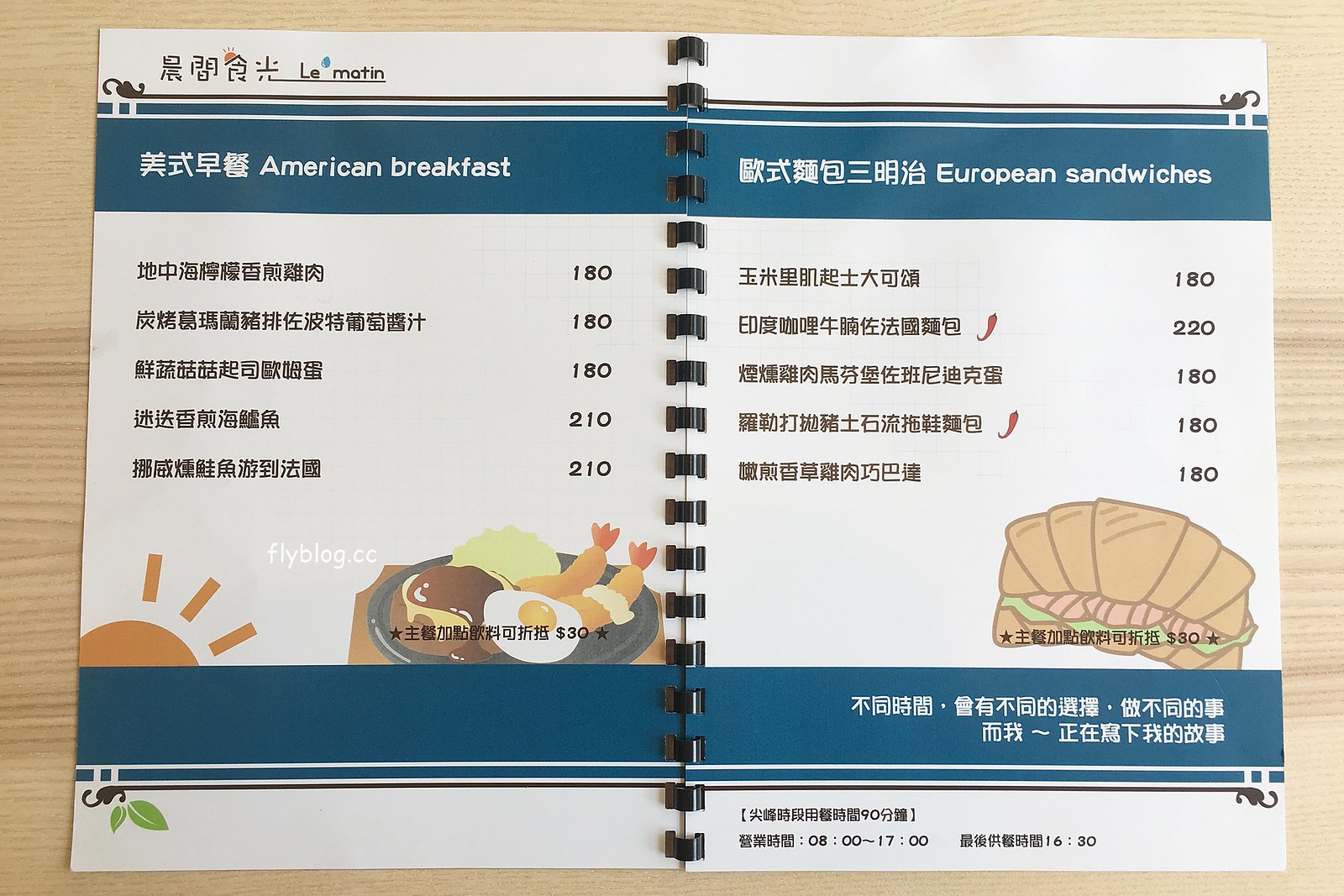The photograph captures a menu laid out on a faux wood grain table or counter. The menu itself is set against a clean, white background. In the upper left corner, there is some Asian script, likely either Chinese or Japanese. Adjacent to this script are the words "La • Metin," where a blue dot separates "La" and "Metin."

On the left page, titled "American Breakfast," there are five breakfast options. Three of these choices are priced at 180, while the bottom two are listed at 210. Beneath the list is an illustration of a sun and a plate of food, which appears to feature eggs, possibly shrimp, and other indiscernible items. This side of the menu is framed by a blue border, and at the very bottom, a white border with two green leaves is visible.

The facing page is titled "European Sandwiches." Similar to the left side, it features a top white border followed by a blue border. Within this blue border is more Asian script along with the text "European Sandwiches." There are five sandwich options; two of them are marked with a chili pepper symbol, indicating they are spicy. The prices for these sandwiches are 180, 220, 180, 180, and 180 respectively. Beneath the list, there is a drawing of a croissant sandwich, another blue border with Asian script, and a final white border at the bottom that includes what appears to be a barcode and some illegible text.